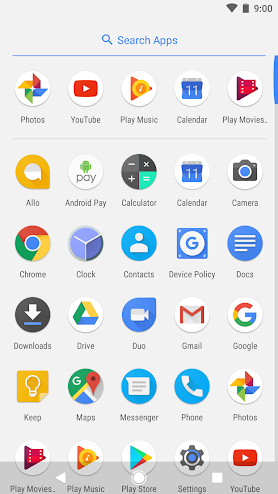This screenshot showcases the app grid on an Android phone. At the top right, the service bar indicates full signal strength, a fully charged battery, and the current time displayed as 9:00. Below this, the search bar at the top provides a convenient way to locate apps.

The apps are neatly categorized, separated by a thin gray line. The top section includes essential apps like Photos, YouTube, Play Music, Calendar, and Play Movies. Below this separator, the apps are listed in alphabetical order, signifying an organized and user-friendly layout.

On the right side, a small blue tab suggests a scrollable interface, indicating that this user has a substantial number of apps, though only those from A to Y are visible on the screen.

The apps visible include Allo, Android Play, Calculator, Calendar, Camera, Chrome, Clock, Contacts, Device Policy, Docs, Downloads, Drive, Duo, Gmail, Google, Keep, Maps, Messenger, Phone, Photos, Play Movies, Play Music, Play Store, Settings, and YouTube. Each app's icon is displayed alongside its name, which is written in unobtrusive, gray-colored text, ensuring a clean and clear visual presentation. Despite the limited screen space, the layout maintains readability and ease of navigation through smaller app icons and text.